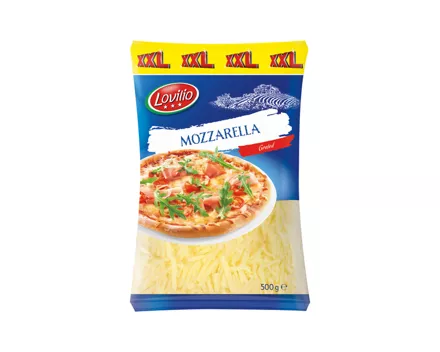This is an image of a package of Lovillo brand mozzarella cheese, distinctly packaged in a bright yellow plastic bag labeled "XXL" in big, bold red letters at the top, indicating it is extra, extra large. Below the yellow section, there is a blue area with a red oval containing the brand name "Lovillo." A white stripe runs diagonally across the middle of the packaging with the word "mozzarella" prominently displayed in blue text. Underneath this text, there is an image showcasing a delicious-looking pizza. The shredded mozzarella cheese inside the bag can be clearly seen through the transparent section of the packaging. In the lower right corner of the bag, it states "500G," indicating the weight of the cheese. The bottom part of the package features additional blue coloring and images, including a picture of pasta, emphasizing the cheese's versatility. The overall design integrates hues of yellow, blue, white, and transparent elements, creating a visually appealing and informative package.